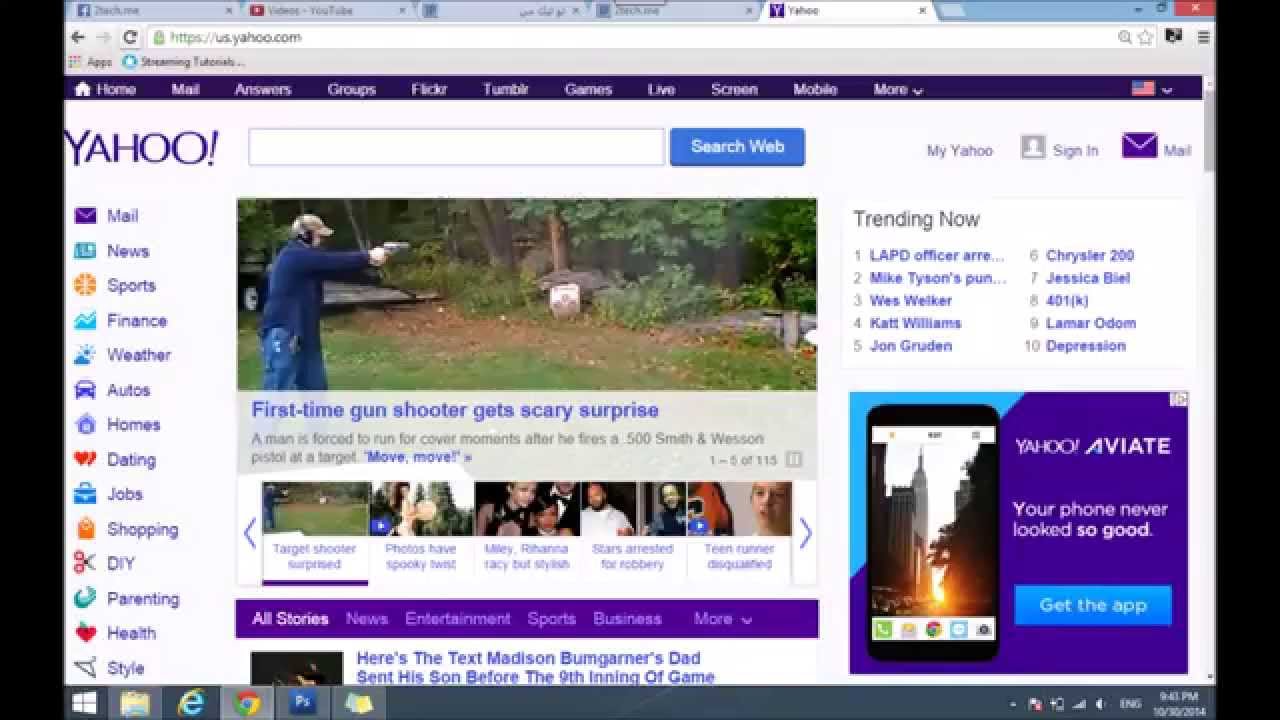Screenshot of a Yahoo Landing Page Displayed in Microsoft Edge Browser

This detailed screenshot showcases the Yahoo landing page as viewed on a Microsoft Edge browser. The open tab clearly indicates it is the Yahoo page, amidst several other tabs.

The Yahoo webpage prominently features a rich purple header with a comprehensive menu bar at the top. The Yahoo logo is situated towards the left side just below the header. Adjacent to the logo, a vertical sidebar lists a variety of Yahoo's features and categories including Mail, News, Sports, Finance, Weather, Autos, Homes, Dating, Jobs, Shopping, Do-It-Yourself, Parenting, Health, and Style.

At the forefront of the main content area, an eye-catching article is highlighted: "First Time Gun Shooter Gets Scary Surprise." Accompanying this headline is an outdoor shooting range photo where a lone individual is captured holding a gun on the left side.

Beneath this leading article, there is a section displaying five articles arranged consecutively in a row. Following this section, another article starts with a purple header encompassing broader categories such as All Stories, News, Entertainment, Sports, Business, and more.

On the far right side of the page, a "Trending Now" box lists about ten trending topics. Directly below this trending section, there is an advertisement for Yahoo Aviate featuring an image of a mobile phone. The ad includes a tagline, "Your phone never looked so good," along with a blue "Get the App" button on the right side.

This layout provides a structured yet dynamic overview of Yahoo's diverse offerings and trending news.